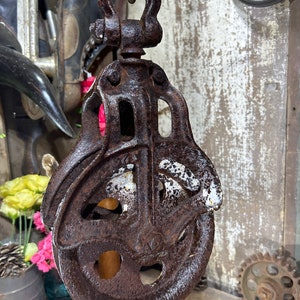This photograph captures a close-up view of an old, rusted metal pulley wheel that looks like it might have originally been silver but has oxidized to a dark brown color. The wheel, which could be a component of a cart or barn door, features five holes around its circumference and is encased in a metal frame secured to a bolt at the top. The backdrop is a weathered, slightly peeling white wooden wall that adds a rustic charm to the scene. A cluster of pink and yellow flowers peeks out from the left side, suggesting this photograph might have been taken outdoors in a garden or tool shed, where the wheel might be artistically placed. Additionally, a slightly rusted cogwheel can be seen resting against the wall in the lower right-hand corner, enhancing the vintage atmosphere of this quaint, curated setting.